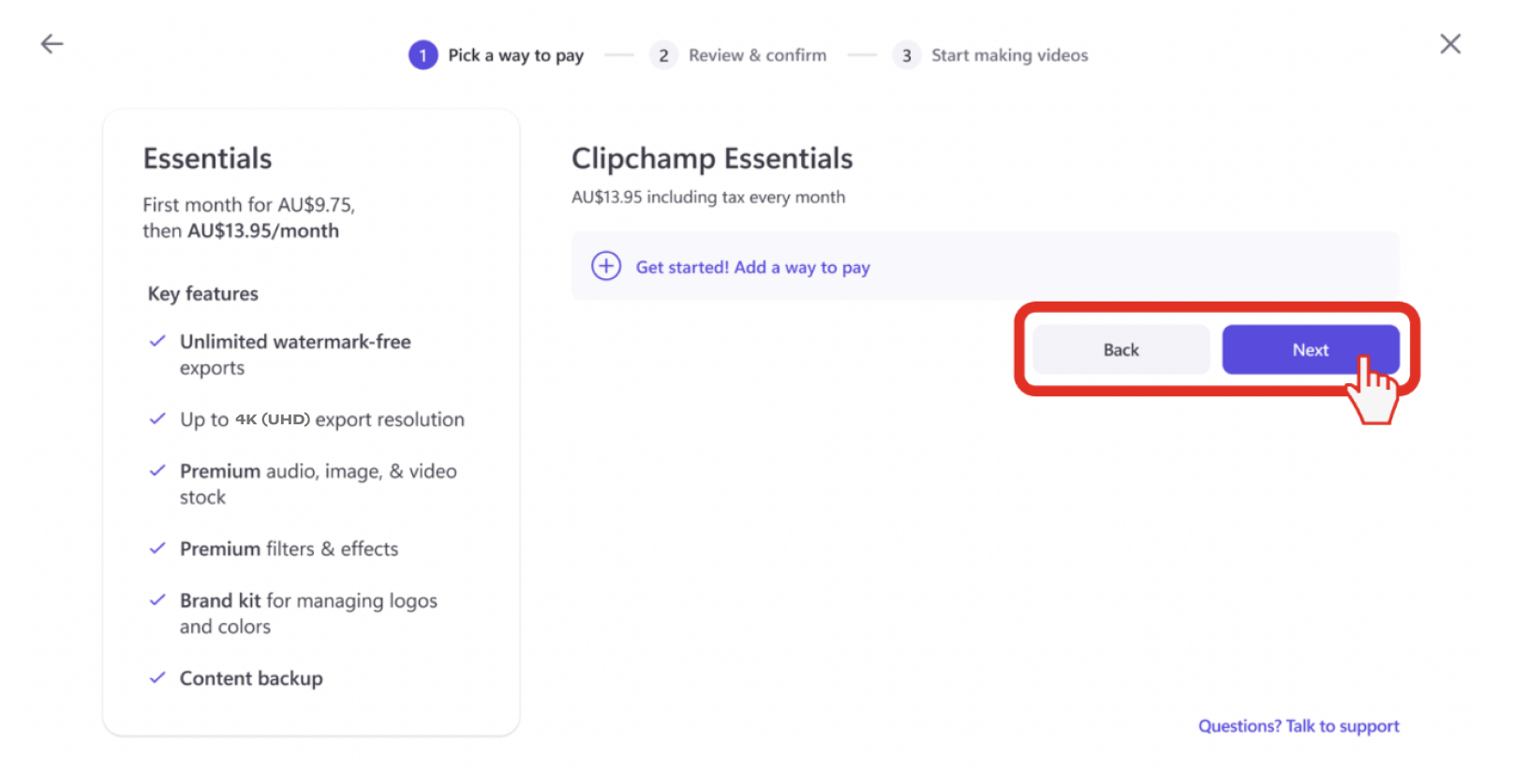In this window, we have Clipchamp Essentials displayed. It is a screenshot featuring navigation buttons: a back button and a next button, which is highlighted in purple with a red circle around it, giving it a cute appearance. The image contains various elements symbolized by words such as "Black," "Gunpowder," and "Hydrazine," arranged around a bullseye. There is also a mention of a price, suggesting a transactional or value-based context. 

A brief narrative illustrates a group preparing for a critical mission, emphasizing the scarcity of their resources: "The rest of our gunpowder won't be able to make any more bullets. Tonight, we need a bomb. We can worry about bullets tomorrow. If we do this and it doesn't work, we'll all be dead tomorrow. Let's make sure it works. To be safe, you need to be at least two inch feet away to make the shot."

A discussion ensues about who will plant the bomb, showcasing a mix of reluctance and determination: "I will." "Won’t pick up a gun, but blowing people up, that you’re okay with?" "We’re blowing up a bridge. There’s not going to be any people on it." The urgency and strategy are palpable as one character insists, "Finn, we have one bomb. We need to use it to kill as many of those bastards as possible. They don’t know we only have one bomb. If we did, why would we waste it on the bridge?" They discuss the concept of deterrence and the impact of perceived strength with historical references, concluding with a poignant thought: "The men who built the A-bombs thought they were peacemakers, too. How’d that work out?"